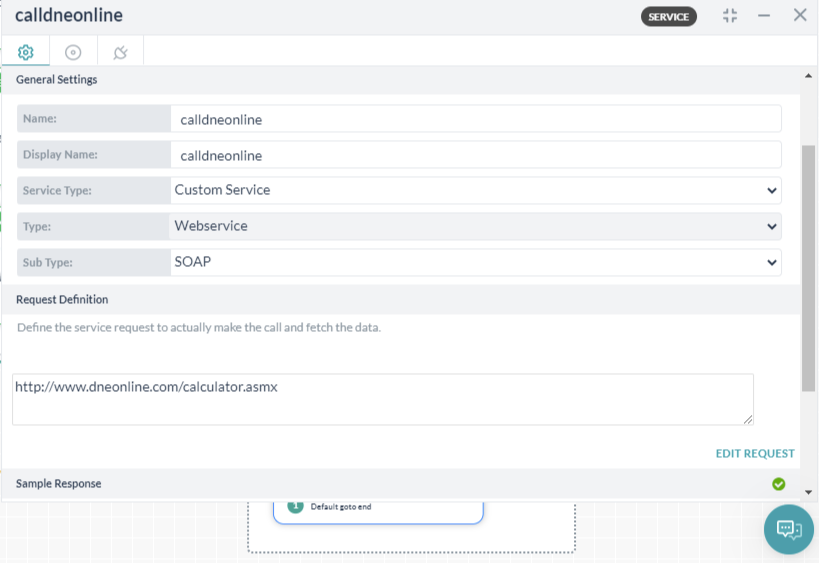This screenshot captures the web interface used for configuring a web service call for a service named "Called and Online." The interface is divided into clearly labeled sections and input fields, presenting a clean and organized layout.

At the top of the interface, the header section contains three buttons for minimize, maximize/restore, and close functions. It also includes a label with the word "Service" enclosed in a black oval, and an icon featuring three horizontal lines, suggesting additional options or settings.

The main configuration area is titled "General Settings," which encompasses several fields for customizing the service. These fields include "Name," "Display Name," "Service Type," "Type," and "Subtype."

Following "General Settings" is the "Request Definition" section. This section contains a text area for defining the service's request URL. The example URL provided is "http://www.dneonline.com/calculator.asmx," signifying access to a web service hosted at "dneonline.com" under the path "calculator.asmx." Below the text area, there is a link labeled "Edit Request," which allows users to modify the request details.

The screenshot also depicts a "Sample Response" section, though it currently does not display any content.

On the left side of the interface, small icons suggest additional settings, enhancing the user's ability to fine-tune the web service call. Overall, the interface is designed to facilitate the configuration and testing of web service calls, offering a user-friendly environment with clearly delineated sections and input fields. It appears to be a reliable tool for the task at hand.